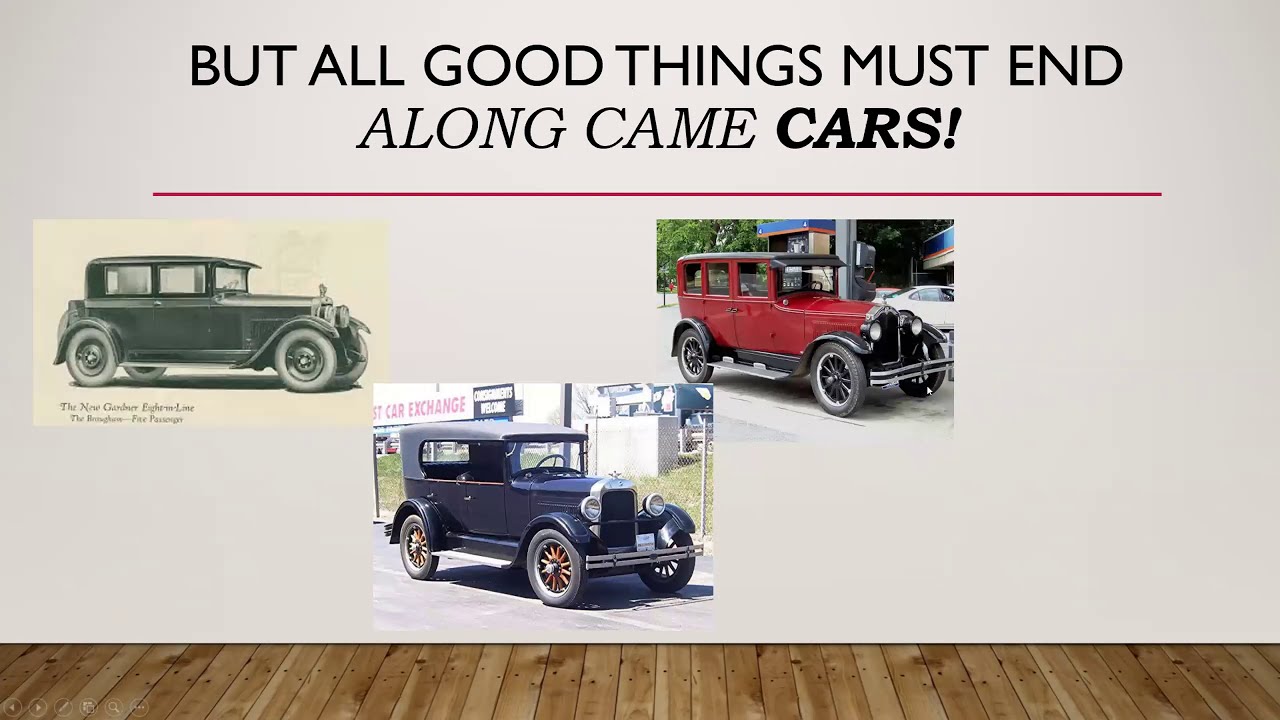The image showcases a white wall and a brown hardwood floor. On the white wall, there is a poster titled "But All Good Things Must End, Along Came Cars," with the word "CARS" emphasized in bold text and a red line below the title. Below the red line, three pictures of antique cars are displayed. The top left image features a black antique car, likely from the Model T era, set against a white background. The middle image presents a blue antique car, positioned against a backdrop that includes a wire fence, a sign, and some buildings, suggesting a modern setting. The top right image depicts a red antique car parked along a roadside in a town, with buildings and a white modern car visible in the background. The poster, which resembles an informational brochure rather than an advertisement, includes small, hard-to-read text likely describing each vehicle.